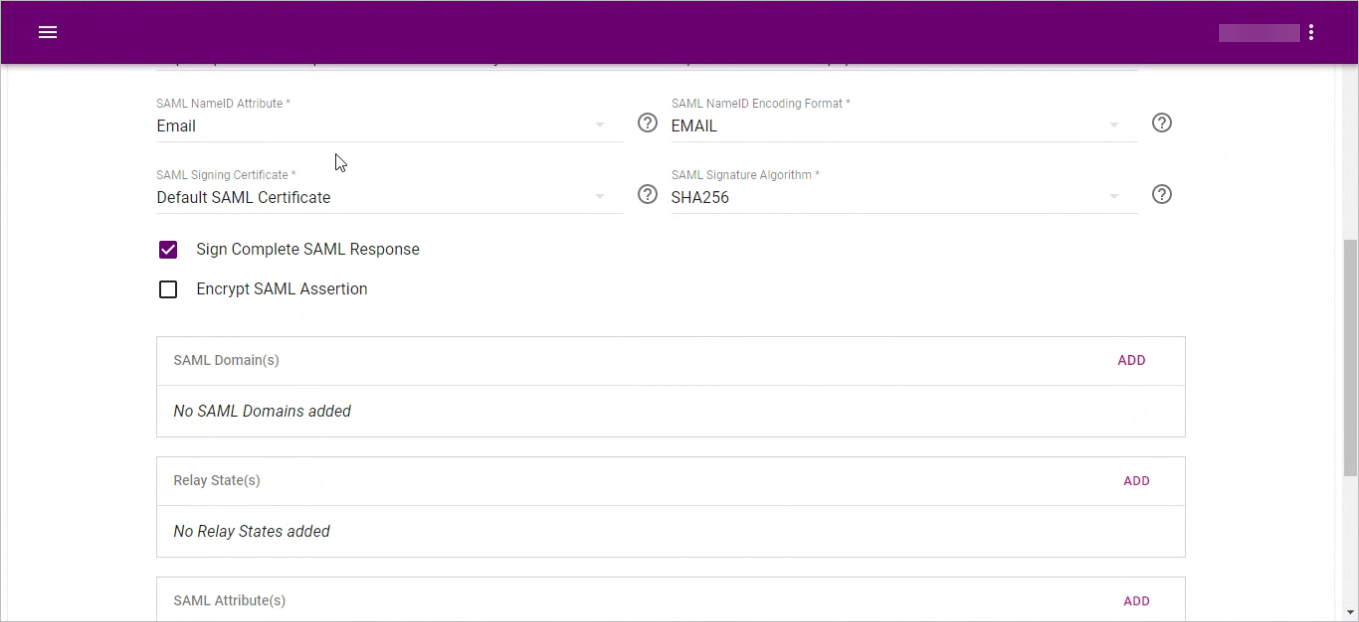A web interface related to SAML (Security Assertion Markup Language) is displayed. The page features a horizontal purple bar at the top, which includes an icon of three horizontal lines stacked on top of each other, indicating a menu. Below this bar, the page has a white background and is organized into several sections for user input. The first section is labeled "SAML Name ID Attribute," with the value "email" entered. Directly beneath this is the "SAML Signing Certificate" field, populated with "default SAML certificate." Following this, there's a section labeled "Sign Complete SAML Response," which includes a filled square with a white checkmark indicating it has been selected. An unchecked option labeled "Encrypt SAML Assertion" follows this. Further down, there appear to be additional fields for entering more information related to SAML configurations.